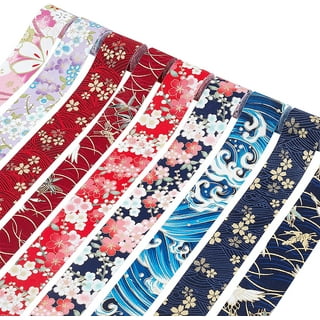The image is a photograph featuring nine distinct rolls of patterned ribbons, meticulously arranged from top left to bottom right against a white background. The ribbons transition from warm to cool colors, beginning with a pink and white floral pattern on the far left. Following this is a purple ribbon adorned with blue and white flowers, succeeded by a red ribbon with white floral designs. Next is another red ribbon that showcases white lines and perhaps hummingbirds. The sequence continues with a red and white ribbon incorporating shades of pink, transitioning to a blue and white floral pattern. Subsequently, there's a ribbon depicting an ocean wave-like design in blue and white. The final two ribbons on the far right are both dark blue; one features white flowers, and the other displays a pattern of white lines and possibly hummingbirds. Each ribbon sports a unique design, predominantly floral, creating a visually cohesive yet varied collection.